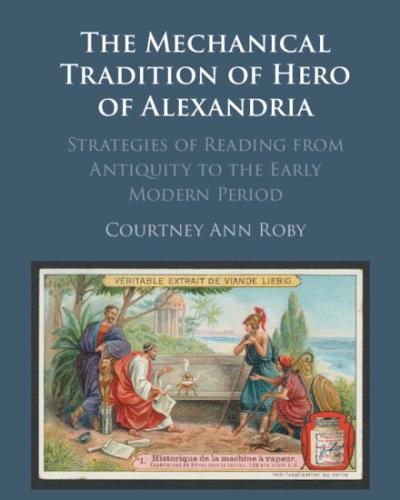This is a detailed description of the book cover of "The Mechanical Tradition of Hero of Alexandria: Strategies of Reading from Antiquity to the Early Modern Period" by Courtney Ann Robey. The cover background is a muted, dark blue with white text for the title prominently centered at the top. Below the title, written in a lighter blue text, is the subtitle, and beneath that, in light white text, is the author's name, Courtney Ann Robey.

The lower half of the cover features a rectangular image depicting an outdoor scene by the ocean. The image shows four individuals from antiquity seated on a beige, arch-shaped bench. The two figures on the left are males; one is dressed in a white robe with a red scarf draped across him, and the other male is bearded and wears no headgear. On the right, there are two women, one of whom seems to lean on a pole or cane. All four are clad in ancient robes, and the scene includes elements like a dome structure, trees, columns, and possibly a statue or shield in the background. The image is bordered in white and black, and contains some Latin text at the top. The intricate details highlight the historical and scholarly nature of the book.